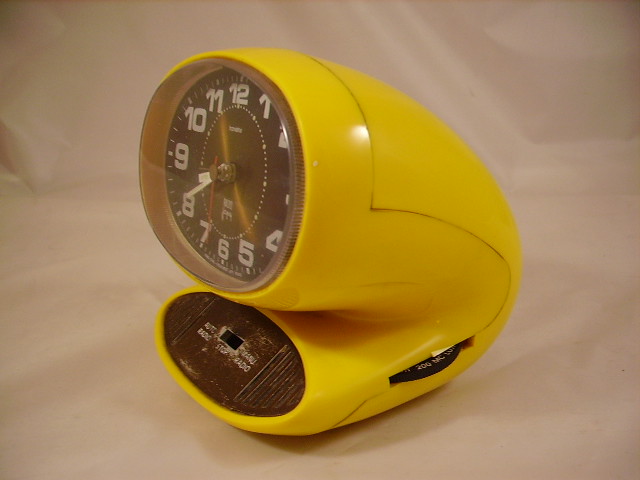In this image, we see a vintage, plastic desk clock, likely from the 1960s to 1990s, with a cylindrical shape folded in half and a bright, yellow exterior. The clock has a black face with white numbers ranging from 1 to 12 and a series of radial markers for the minutes. The hour and minute hands are white, while the red second hand and another white hand, presumably for setting the alarm, add a contrasting visual detail. On the right-hand side of the clock, there is a small black radial dial, possibly for setting the alarm or tuning the radio. Below the clock face, there's a black switch likely used to activate or deactivate the alarm function. Additionally, the bottom part of the clock features dark brown decor with some lettering about the radio functionality. Positioned on a beige or white cloth background, this clock, with its dual functionality as an alarm and perhaps a radio, suggests a nostalgic feel with its toy-like appearance and old-fashioned design.